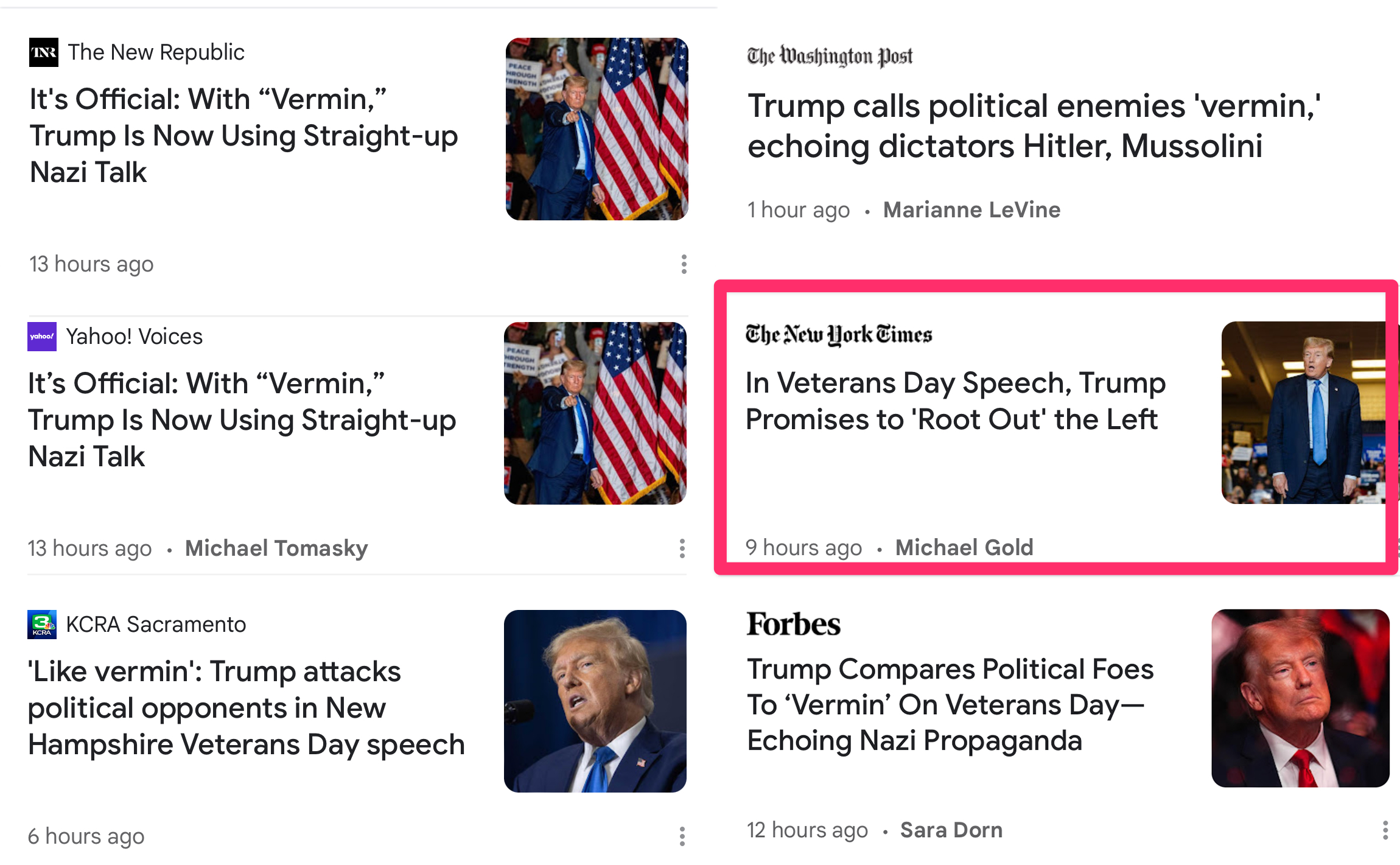The image showcases a collage of headlines from various newspapers, alongside multiple photographs of former President Donald Trump. The first headline, from The New Republic, declares: "It's official with Vermont: Trump is now using straight-up Nazi talk," accompanied by an image of Trump standing by an American flag. The Washington Post's headline reads: "Trump calls political enemies 'vermin', echoing dictators Hitler and Mussolini," while another headline from Yahoo Voices mirrors The New Republic’s claim about Trump’s rhetoric in Vermont.

Another headline from KCRA Sacramento states, "Like 'vermin': Trump attacks political opponents in New Hampshire Veterans Day speech," with a corresponding photo of Trump, clad in a blue suit and a shiny royal blue tie, seemingly at the speech. Additionally, an image outlined in red shows Trump with his back to an audience, possibly addressing a crowd on a round stage, paired with a New York Times headline: "In Veterans Day speech, Trump promises to root out the left." The final headline at the bottom, depicting Trump sitting and intently listening or focusing, is from an undisclosed source and reads: "Trump compares political foes to 'vermin' on Veterans Day, echoing Nazi propaganda."

Each headline and image collectively underscore the recurrent theme of Trump's inflammatory rhetoric, drawing parallels with notorious historical figures.